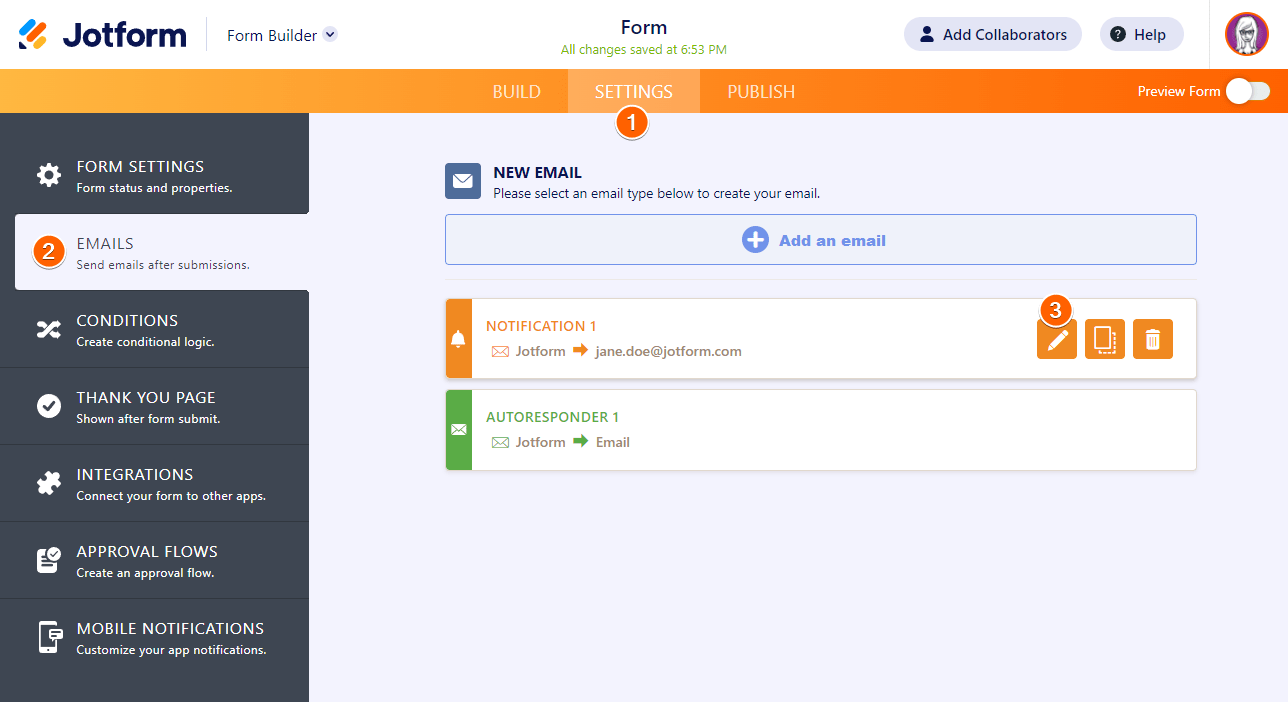This screenshot displays a webpage from the website "JotForm." At the top of the page, there is an orange navigation bar featuring three white-lettered options: "Build," "Settings," and "Publish." The "Settings" option is highlighted in a lighter shade of orange. Below this, there is a prompt to "Add a New Email."

The left sidebar, colored in dark grey, presents a vertical menu of options. These options include "Form Settings," "Emails," "Conditions," "Thank You Page," "Integrations," "Approval Flows," and "Mobile Notifications." Both the "Settings" and "Emails" options are highlighted. Next to "Settings," the number one is displayed, while the number two is shown beside "Emails." Additionally, the number three is indicated above an icon located on the right side of the email section.

The overall interface reveal the structured steps suggested by the numbered indicators, potentially guiding the user through a setup or configuration process.